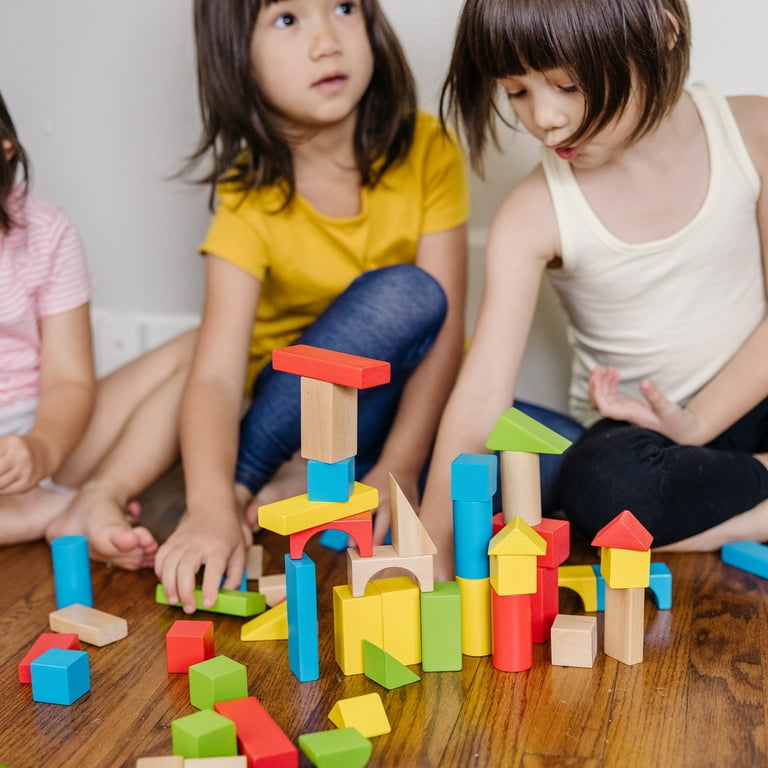In a cozy, indoor preschool room painted with grey walls and white trim, three young girls, all around four years old, are seated on a polished wooden floor, immersed in play. The room seems well-suited for their activities, featuring an array of colorful building blocks, including red, blue, green, yellow, and natural wood tones. The girl on the right wears a white tank top and black leggings, her brown hair neatly styled with bangs and falling to her shoulders. Next to her, another girl dons a yellow short-sleeve shirt paired with blue jean-like leggings, her brown hair reaching her shoulders as well, suggesting they might be twins. Partially visible on the left is another girl in a pink and white striped shirt and gray shorts, her brown hair slightly shorter than the others. The vivid scene captures the innocence and creativity of their early years as they engage with their toys on the warm, brown floor.